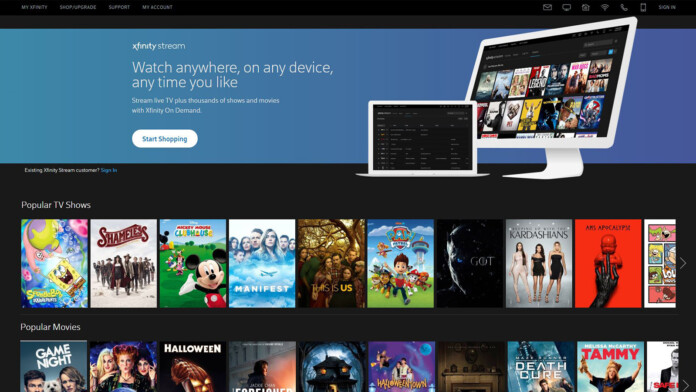**Caption:** 

On a vibrant blue background, "Xfinity Stream" is displayed in clean, small white text at the top. Beneath this, the service's promise is stated: "Watch anywhere, on any device, anytime you like." Centrally located is a horizontally placed white oval button labeled "Start Shopping." 

To the right, a high-resolution laptop screen showcases the streaming interface. Below the laptop, a sleek white handle adds a touch of modern design. 

The laptop screen is filled with enticing movie covers arranged in two rows. Below the image, the text "Popular TV Shows" introduces a selection of hits. First is "SpongeBob SquarePants," with the friendly yellow sponge and his best friend, Patrick Star, in his signature pink starfish form and colorful shorts. Next to it are "Shameless," "Mickey Mouse Clubhouse," "Manifest," and "The Kardashians." The show "AHS Apocalypse" stands out with its striking bold red design and an ominous black leather hand emerging from the bottom.

The second row features popular movies, starting with "Game Night," followed by the Halloween classics "Hocus Pocus" and "Halloween." Next is "Death Club," and finally, the comedy "Tammy." Each image is crisp and vibrant, drawing attention to the diverse array of entertainment options available.